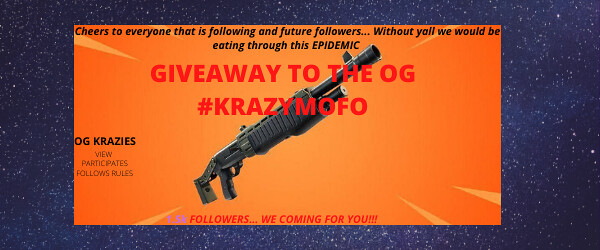**Event Poster for Online Giveaway**

The poster has a dark blue background adorned with scattered white dots, giving it a starry night appearance. It is designed in a landscape format to capture attention. At the center of this backdrop is an orange rectangular box, which adds a vibrant contrast to the blue background.

Inside the orange box, the central feature is the headline "Giveaway to the OG" in large, red, bold fonts that immediately draw the eye. Below the headline is a prominent image of a gun, placed right at the center. At the bottom center of this rectangular box, there's another image of a gun, creating a symmetrical visual balance.

In the top left-hand corner of the poster, there is the text "OG Crazies" followed by instructions for participation: "If you participate following rules." Overlaying the entire image at the top is a tagline in smaller font: "Cheers to everyone that is following and future followers. Without y'all we would be eating through this EPIDEMIC," with the word "EPIDEMIC" emphasized in all capital letters.

Additionally, the poster displays a celebratory note with the text: "1.5k followers. We are coming for you," hinting at the growing community and the excitement surrounding the event. The mention of "#CrazyMofo" at the center under the headline serves as a hashtag for social media engagement, further binding the community together.

Overall, the poster effectively conveys the event details with a visually engaging design and clear messaging for an online giveaway event.